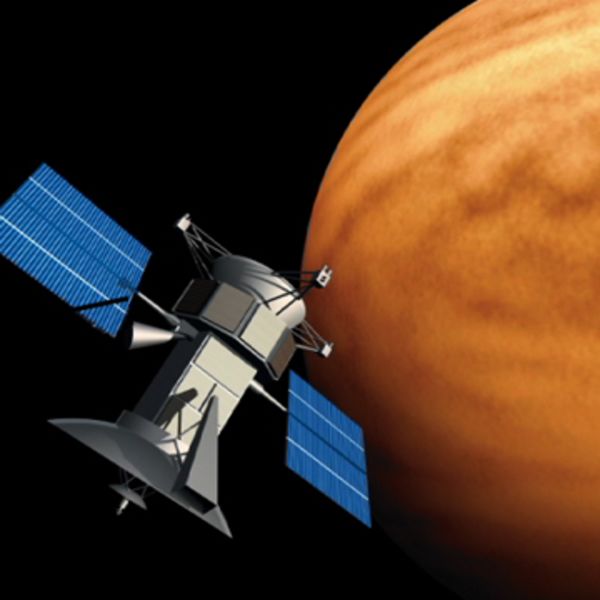The image depicts a computer-generated scene of a space probe orbiting a planet that is reminiscent of Mars, displaying a reddish-brown and tan surface with cloud formations. The probe, positioned in the lower left of the image, features a white cylindrical body flanked by two solar panels angled toward the light source in the upper right to power the device. The cylindrical body is somewhat plunger-like in shape, with various antennas and cables extending from it. Its main antenna points downward. To the top right of the image, just under half of the planet is visible against the black backdrop of space, devoid of stars. This artistic representation lacks identifying markings indicating the probe's origin, emphasizing its generic design as it orbits in deep space.